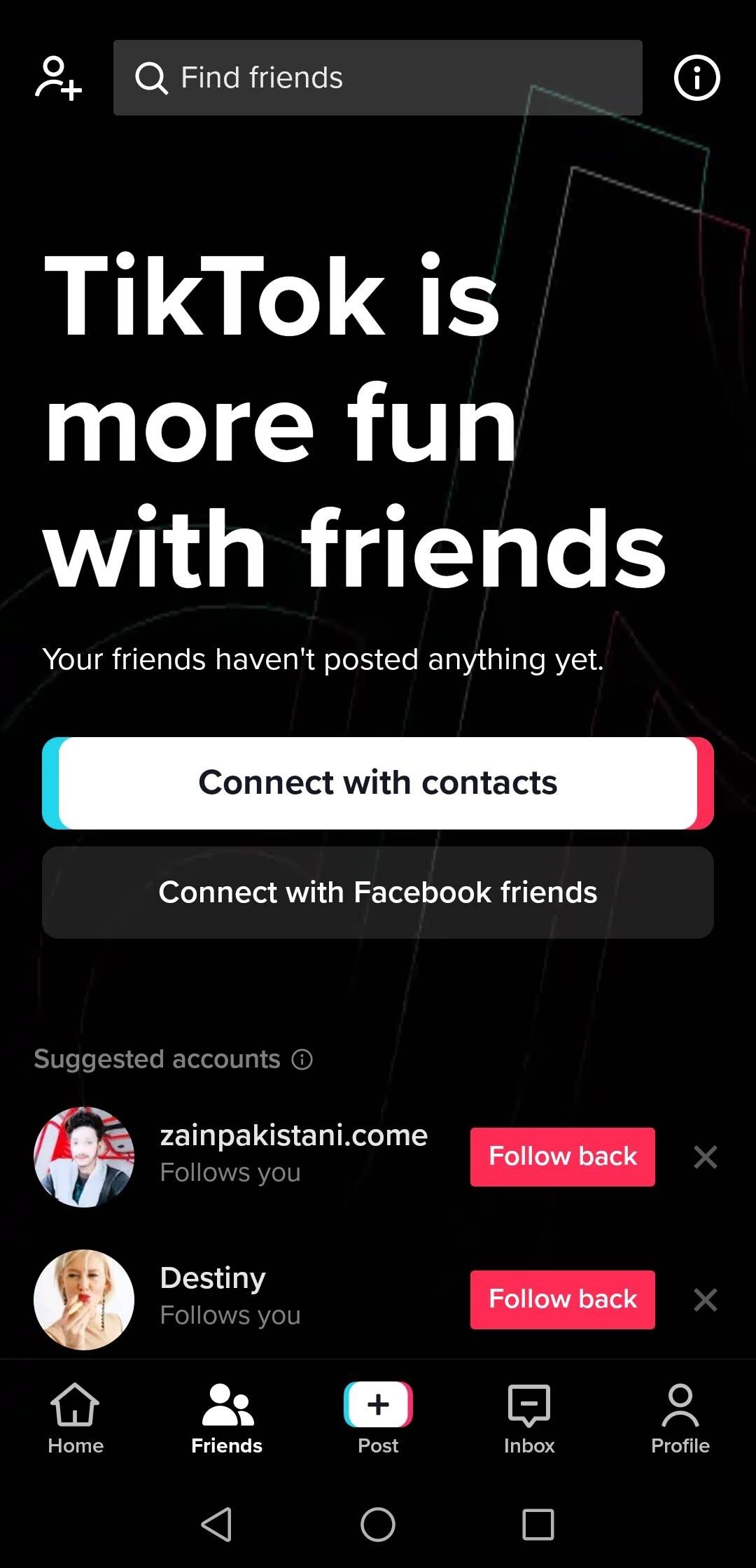The image is a screenshot taken from a mobile device displaying the Friends page on the TikTok app. The vertical layout of the screenshot confirms it was captured from a smartphone. At the bottom of the screen, the device's navigation bar is visible, featuring icons such as a sideways triangle, a circle, and a square, indicative of typical mobile navigation buttons.

Above this, TikTok's own menu bar is clearly displayed, comprising five main options from left to right: Home, Friends, Post, Inbox, and Profile. The "Friends" icon is highlighted, indicating that the user is currently on the Friends page.

In the main content area, the app suggests two accounts for the user to follow back. The first suggestion features a profile picture of a male with curly hair against a red and white background, under the username "zainpakistani.com." This account follows the user, and there's a "Follow Back" button next to it. The second suggestion displays a female with blonde hair, named "Destiny," who also follows the user, accompanied by a similar "Follow Back" option.

At the top of the screen, a banner message reads, "TikTok is more fun with friends." Below this, it states, "Your friends haven't posted anything yet," and offers two prompts for connecting with friends: "Connect with Contacts" and "Connect with Facebook Friends."